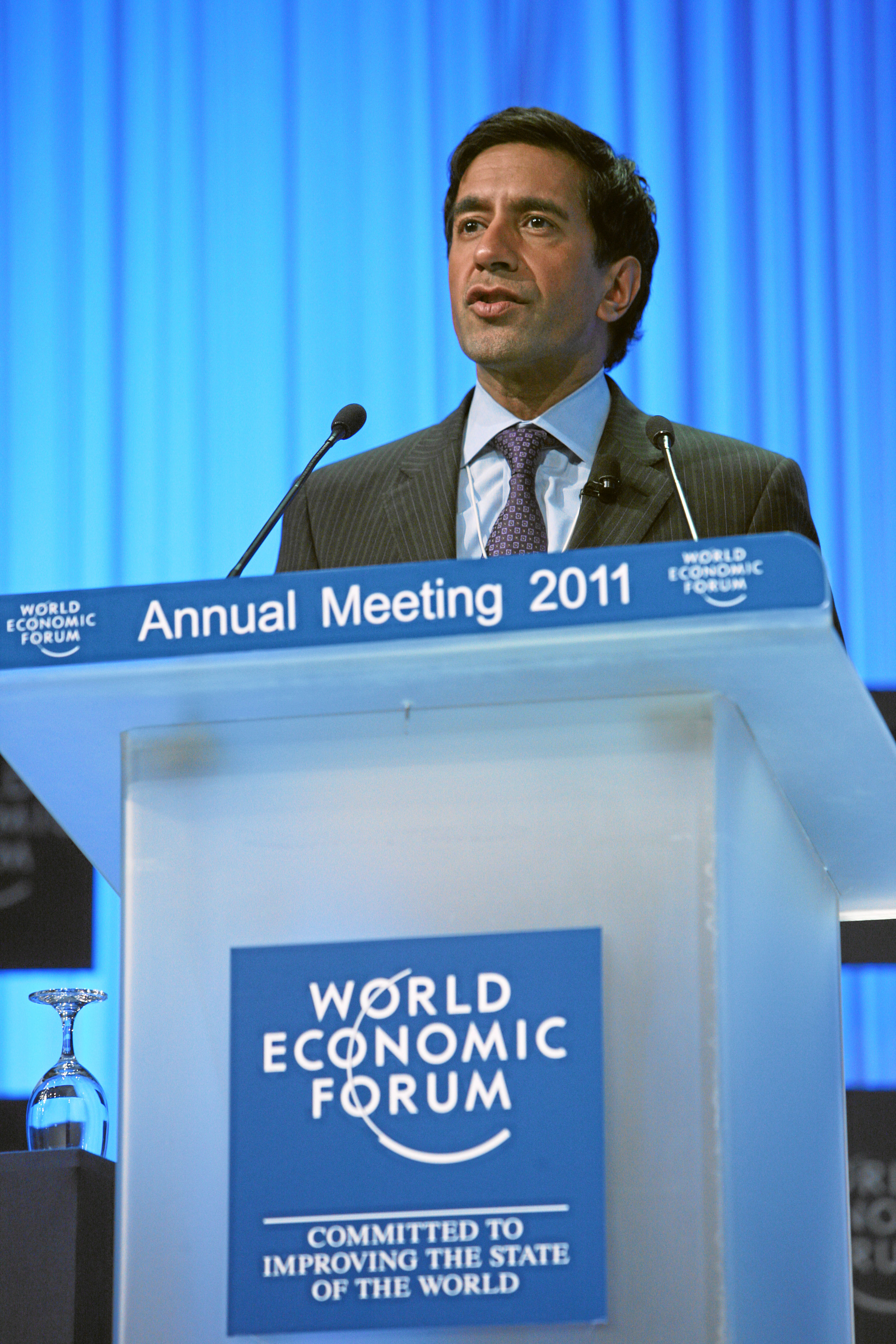This vertical image captures a man speaking at the World Economic Forum Annual Meeting 2011, as indicated by the text at the top of the glass podium. The main logo of the forum is centrally located on the podium in a striking blue, beneath which it reads, "Committed to Improving the State of the World." The speaker, who appears to be of Southeast Asian descent, has short, thick black hair and is dressed in a pinstripe black suit, paired with a light blue shirt and a muted purple geometric tie. He speaks into two microphones extending from the podium, with an additional microphone clipped to his left lapel. The backdrop features a light blue curtain contrasting the dark blue of the logo. Just below and to his right, there is a table with an upside-down wine glass, likely serving as a water glass. The image is well-lit and captures a serious yet optimistic atmosphere.